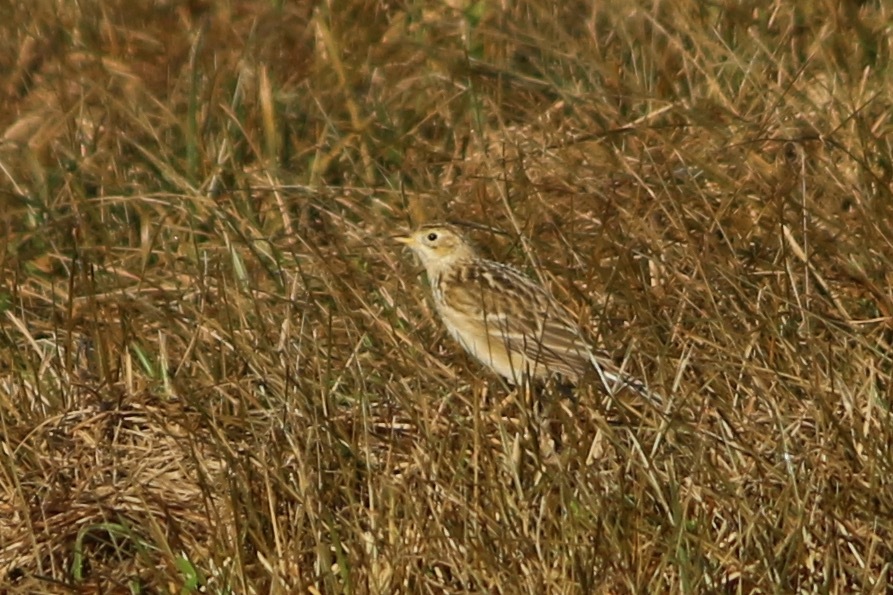The image showcases a small bird standing on the ground amidst a patch of dark green and predominantly brown grass, indicative of a heat wave or drought. The bird is positioned almost centrally but slightly to the right and gazes leftward in profile. It blends seamlessly with its surroundings due to its camouflaging plumage. The bird's upper parts, including its wings, feature a mixture of dark brown, light brown, and tan hues, while its cheeks and face are lighter. The throat and belly are a much lighter, off-white color. Its small beak is a dull yellow, and one black eye is visible facing the camera. Despite some grass obscuring it, the bird's tail appears a bit darker with what seems like a black line. The horizontal composition of the image is wider than it is tall, with the bird almost vertically centered from top to bottom.